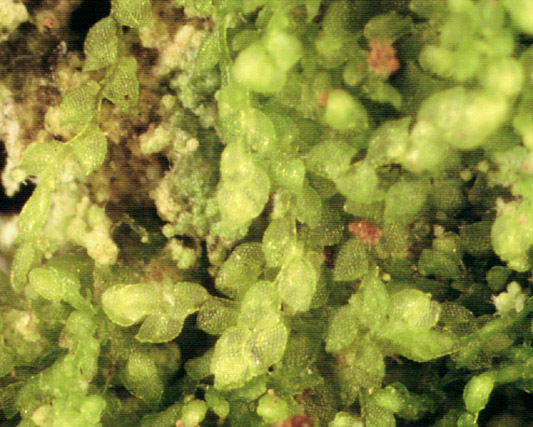The photograph appears to be a highly magnified, slightly blurry image of a plant, possibly viewed under a microscope. The foreground is dominated by many light green and dark green oval or circular leaves, each with visible veins running through them. Scattered throughout the image are hints of orange and yellow colors, which might suggest the presence of fruit or berries on the plant. The overall grainy texture adds to the difficulty in precisely identifying the subject, but the predominant features are clearly the magnified, veined green leaves.